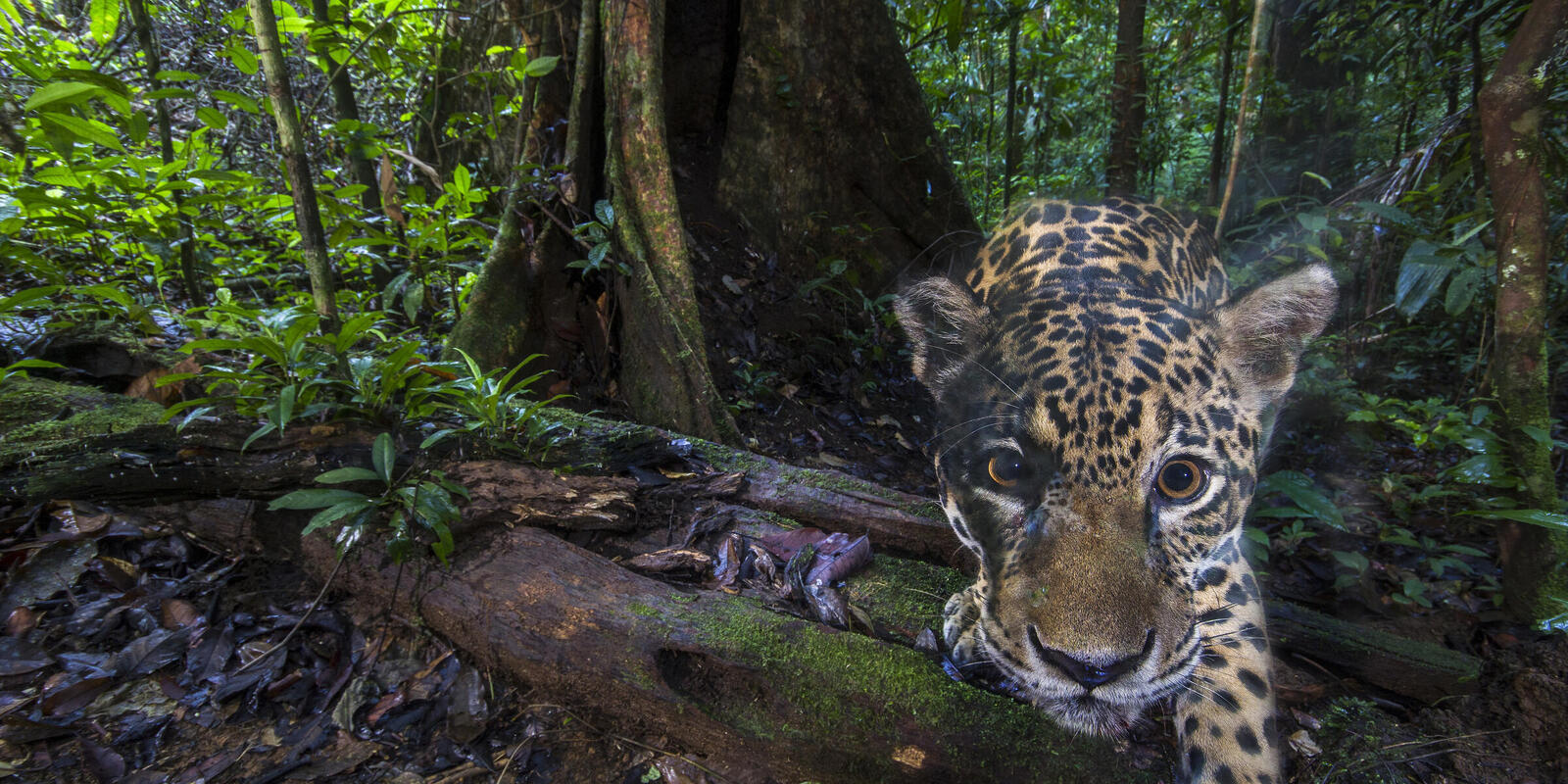In this striking and highly detailed photograph, a curious leopard is captured approaching the camera in a tropical rainforest. With wide, dilated eyes that stand out as big black circles, the leopard's face dominates the scene, its left paw visible underneath the camera lens as if investigating the device. Positioned about a third of the way from the right side of the frame, the majestic animal is highlighted against a lush backdrop of greenery. A large tree trunk lies directly behind the leopard to the left, surrounded by an abundance of smaller trees, bamboo, and other forest foliage. The ground in the bottom left corner appears wet, hinting at the moist, tropical environment that envelops the scene. These combined elements create a captivating snapshot that melds the grace of the leopard with the wild beauty of its jungle habitat.